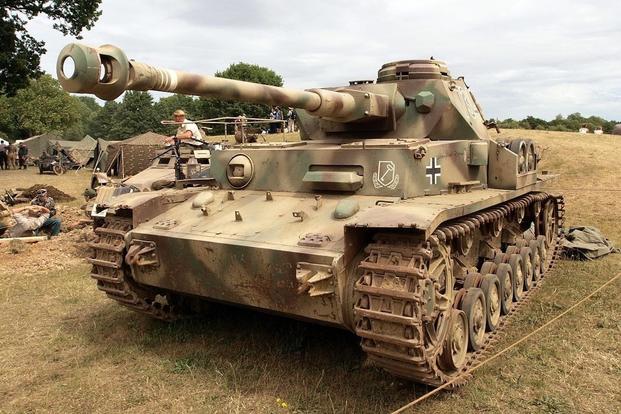The image features a camouflage-painted World War II German Tiger tank positioned in a flat, grassy terrain with low, clipped grass. The tank is adorned with a distinctive cross emblem on its side and a large central gun, with visible tracks and retrofitted features suggesting an upgrade. The tank is roped off, indicating a display set up perhaps for visitors or historical exhibitions. 

To the right, a man dressed in army fatigues sits atop a brown military vehicle different from the tank. Further in the background, there are several tents, likely resembling army tents, with people gathered around them. Among them, a man in a white shirt is noticeable, along with others who seem to be sitting and interacting in the distance. Beyond the tents, a dense line of trees marks the horizon, flanked by a cloudy sky with grayish-white clouds, suggesting overcast weather yet not indicative of impending rain. The overall scene conveys a historical or commemorative setting, possibly depicting a wartime reenactment or display.